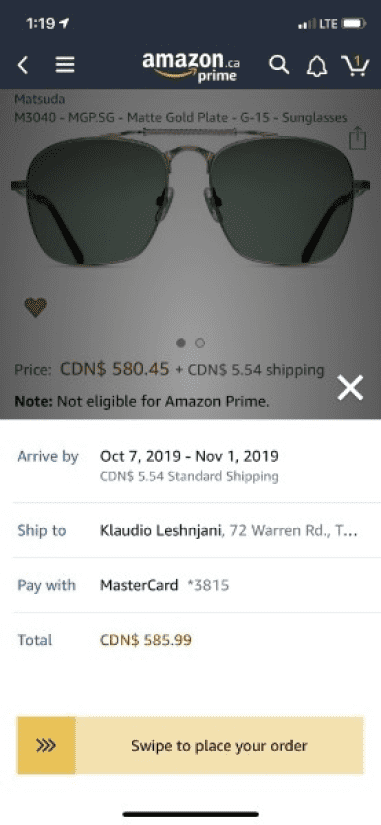This detailed caption describes a screenshot of the Amazon Prime shopping interface on a cell phone:

At the top center, the Amazon.ca Prime logo is prominently displayed. To the left of the logo, there is a back arrow, and to the right, three horizontal lines symbolizing the menu. Following the logo to the right, there are icons for search, notifications (bell), and the cart, which indicates one item inside.

The background features an image of sunglasses by "Mitsuda," with the model number "M3040-MGP5G" and the description "Matte Gold Plate G15 Sunglasses." Below the label is a photo of the stylish sunglasses, accompanied by a heart icon for adding them to the wishlist on the left.

The price of the sunglasses is displayed in yellow text as CAD $580.45, with an additional shipping cost of CAD $5.54. A note beneath this price informs that the item is not eligible for Amazon Prime. Further down, delivery details state the estimated arrival date as between October 7, 2019, and November 1, 2019. The item will be shipped to Claudio L., with the address "72 Warren Road." Below this, the payment method is listed as MasterCard ending in 3815, with a total cost of CAD $585.99.

At the bottom of the screen is a conspicuous yellow bar with the instruction to "Swipe to place your order."